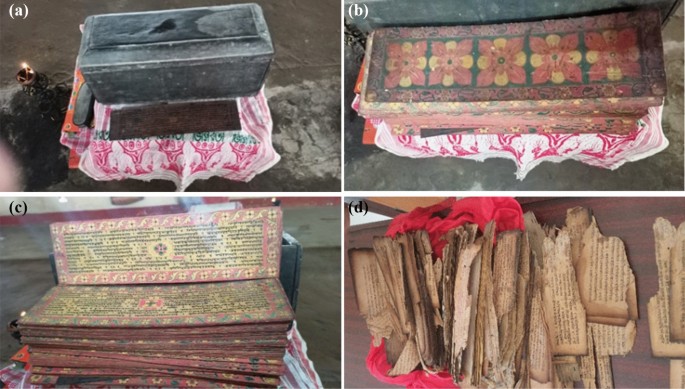The image depicts a collage of four photographs labeled A, B, C, and D, each situated in one of the four corners over a white backdrop. The labels appear in lowercase letters with parentheses around them: 'a' in the upper left, 'b' in the upper right, 'c' in the lower left, and 'd' in the lower right. 

In photo A, situated in the top left corner, there’s an image of what seems to be a black stone case resting on a white powdery or sandy surface, possibly cement. This case may suggest a protective box or container for the items in the subsequent photographs.

Photo B, in the upper right corner, appears to display a set of old papers or documents, intricately lined with printed flower designs. These papers seem to have been carefully laid out, indicating their historical or delicate nature.

Photo C, in the lower left corner, shows several rectangular pieces that resemble old papers or booklets, neatly stacked on top of one another. The papers are colorful, featuring hues of blue, green, and yellow, with writing that might be in Arabic or Hebrew, although the text is not clearly legible.

In photo D, located in the lower right corner, there is a collection of tattered and possibly burnt pieces of paper scattered over a wooden backdrop, with one piece resting on a red cloth garment. These fragmented pieces appear to be remnants or salvaged parts of a once intact document or book.

Together, the series of photographs appear to document the discovery and condition of historical artifacts, specifically old papers that may have been recovered from the black case shown in photo A. The sequence suggests a narrative of preservation or a timeline of use and damage associated with these aged documents.